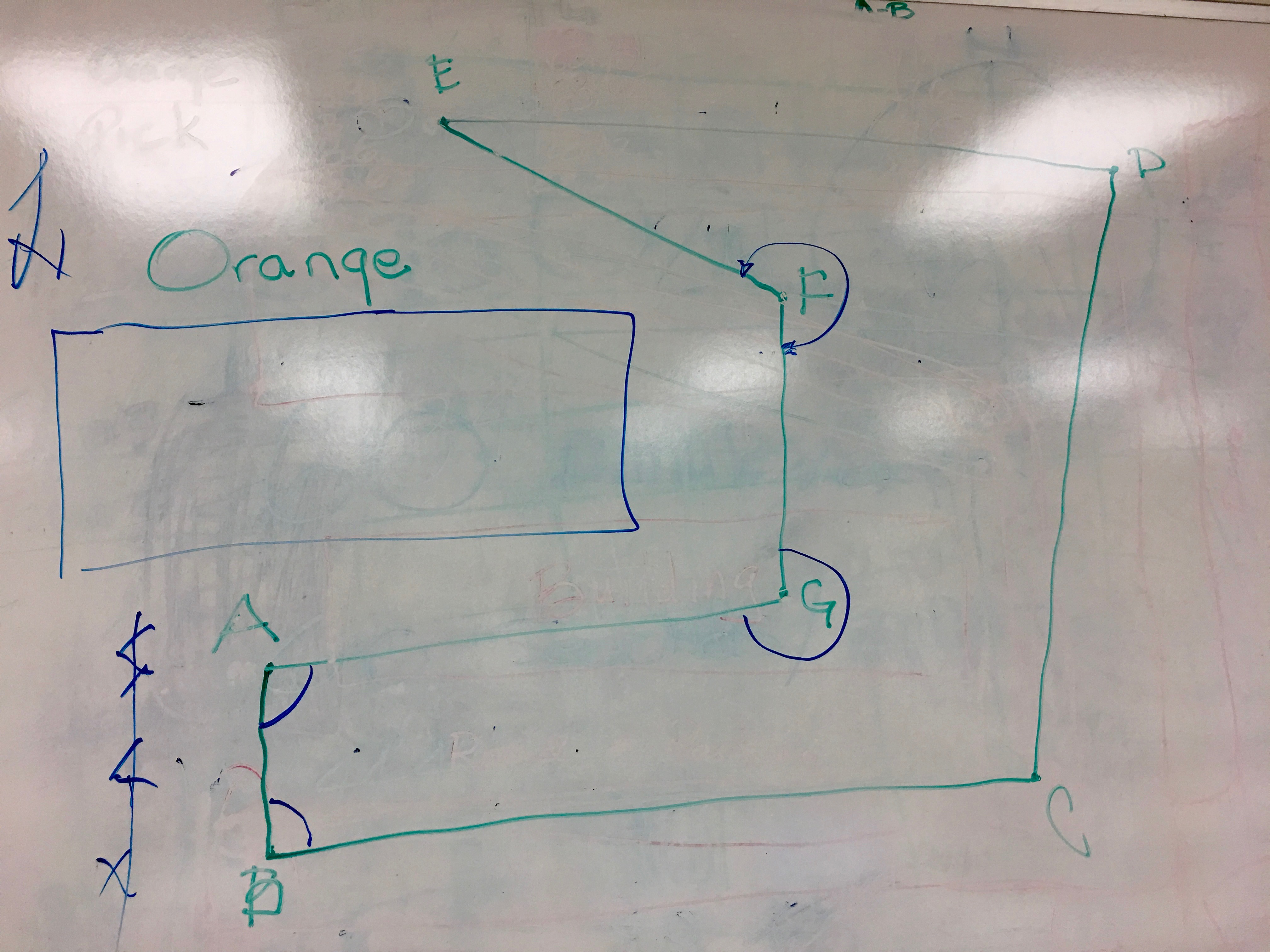In this image, there is a whiteboard that appears to have been used repeatedly, obscuring some parts of the present drawing due to multiple erasures. The whiteboard contains a rather complex, possibly mathematical diagram primarily composed of various geometric shapes and labeled sections.

At the bottom of the diagram, there is a sequence of labels starting with "C", followed by "A", "B". These labels correspond to different parts of the shapes drawn on the board. There is a smaller rectangle that transitions into a larger rectangle extending upwards. On one side, this larger rectangle has a pointed section, indicating a specific area where label "A" is located.

The diagram also features multiple diagonal lines. One such diagonal, specifically at label "B", is prominently outlined. Circling these elements, the labels proceed as "C" on the outer part, followed by "D" and "E".

Within the rectangle, there are two half-circles labeled "F" and "G" respectively. Above these, the word "orange" is seen, although interestingly, the portion labeled "orange" is actually colored green. The diagonal lines within the diagram are drawn with a blue marker, while the majority of the other elements are depicted in green marker. 

This intricately detailed diagram on a heavily-used whiteboard seems to convey a layered and coded spatial relationship between the labeled sections and their corresponding shapes and lines.